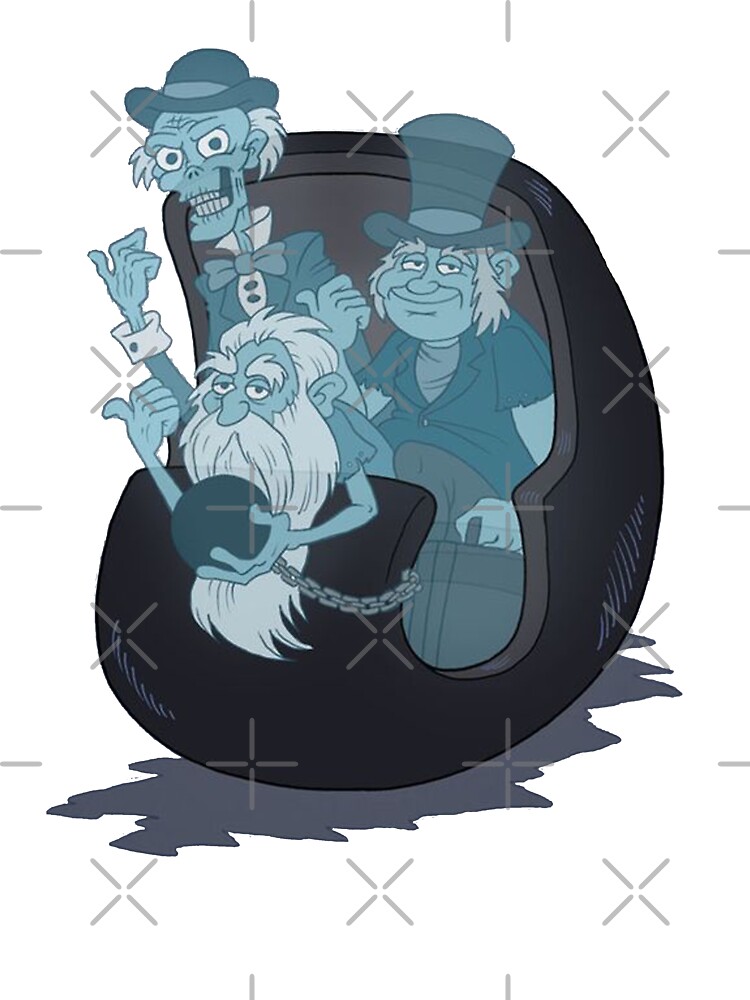This detailed cartoon image depicts three ghostly, translucent, light turquoise figures sitting in a black, egg-shaped cart resembling an amusement park ride vehicle. The background is solid white, covered with scattered gray X's and dashes.

In the back left seat is a skeleton adorned with a top hat, bulging eyes, raggedy clothes, and a bow tie. To the right is a character with long gray hair, smiling under a taller top hat, wearing a short-sleeved shirt and brown pants. The front seat is occupied by an older man with thick, shaggy eyebrows, a long gray beard, and equally bushy hair. He holds a ball and chain, appearing connected to it, and all three characters have their thumbs out, giving a hitchhiking gesture. The vehicle has a dark shadow underneath.